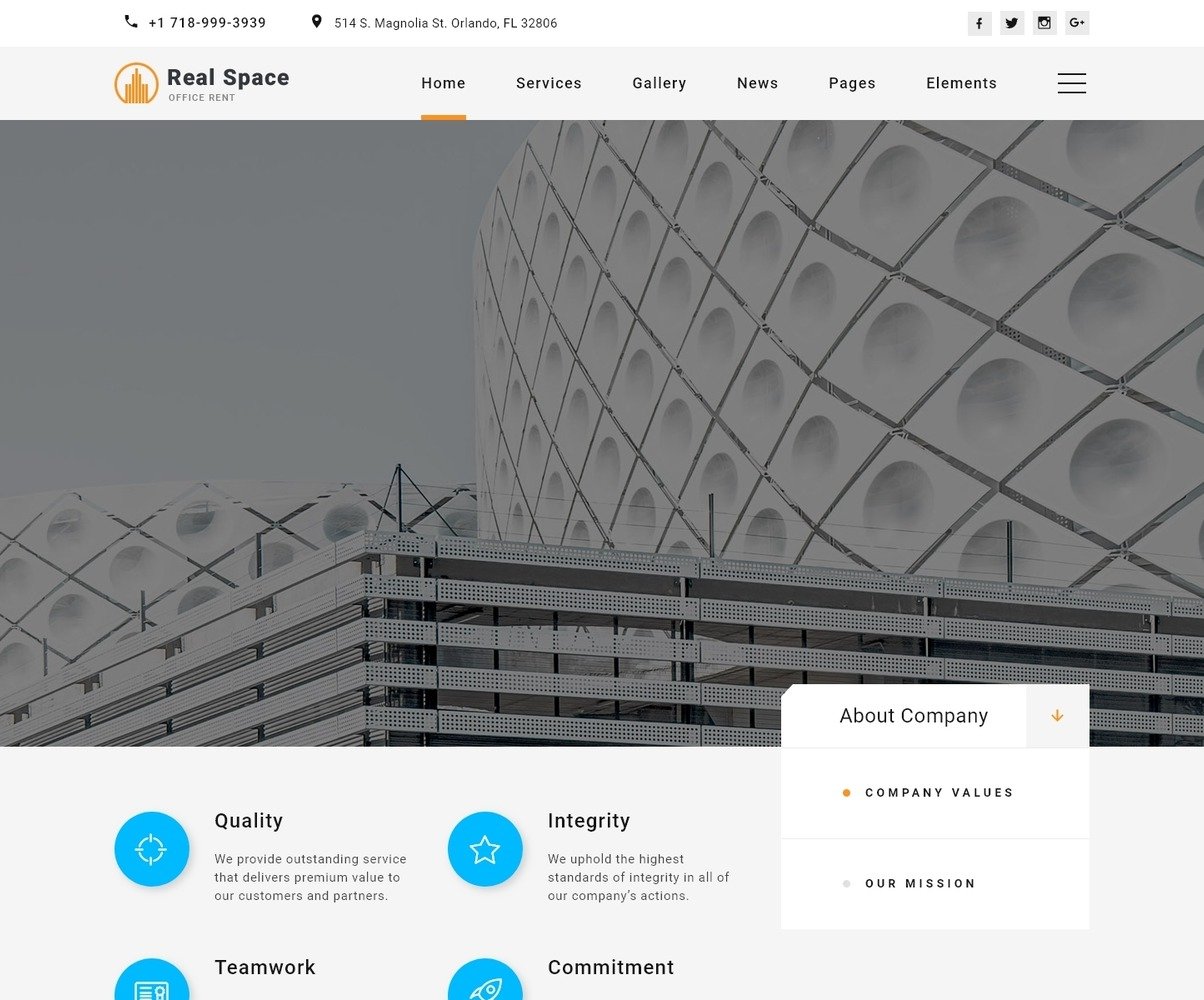A detailed web page screenshot featuring a contact and location header, a robust menu, and detailed company values. At the top, a phone icon displays the number +1 718-993-939, and a location icon indicates the address 514 South Magnolia Street, Orlando, Florida, 32806. To the right, social media icons for Facebook, Twitter, Google Plus, and Instagram are visible. The gray menu bar adorned with the "Real Space" logo and "Office Rent" has several navigation items: Home (highlighted with an orange bar), Services, Gallery, News, Pages, Elements, and a Hamburger Menu.

Below, a large photograph of a multi-story building with a unique, almost golf ball-like structure dominates the page. At the bottom left, a table with blue icons illustrates key company values: 

1. **Quality:** "We provide outstanding service that delivers premium value to our customers and partners."
2. **Integrity:** "We uphold the highest standards of integrity in all of our company's actions."
3. **Teamwork:** Followed by 
4. **Commitment:** (text cut off)

A white box floating over to the right contains headings "About Company," "Company Values," and "Our Mission."